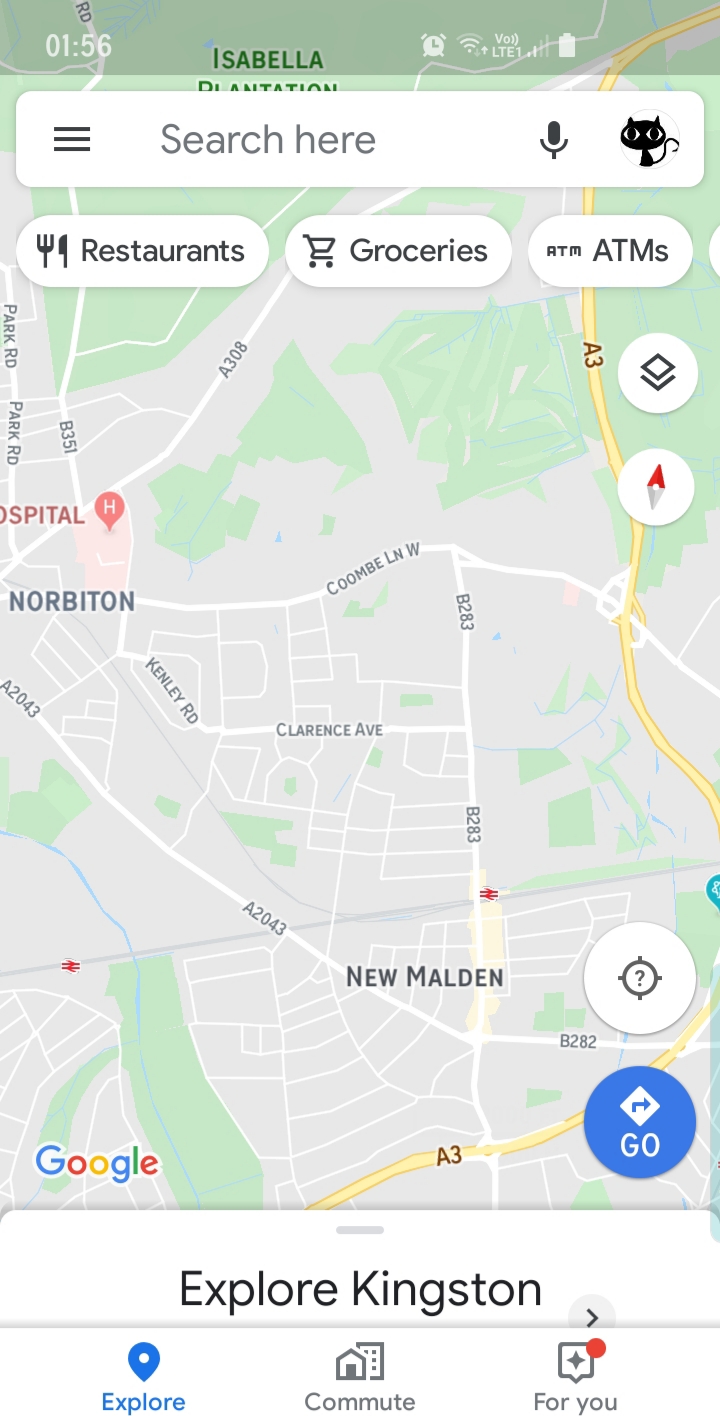The image displayed on a smartphone screen shows the current time as 1:56, with the battery fully charged and a strong network connection. At the top, there is a search bar labeled "Search here," which also includes a microphone icon for voice search. To the left of the search bar are three horizontal lines indicating a menu. On the same top bar, there are options for "Restaurants," "Groceries," and "ATMs."

Below the search bar is a digital map interface, seemingly a road map. Key points of interest are marked on the map, including a hospital indicated by a red pin with an 'H', and towns labeled "Norbiton" and "New Malden."

At the bottom of the map, there is a blue circular button labeled "Go," which incorporates a diamond-shaped icon with an arrow. Above this button, there is a compass symbol containing a question mark.

The map and interface are provided by Google, evidenced by the Google logo in the lower left corner, featuring the familiar blue 'G', red 'O', yellow 'O', blue 'G', green 'L', and red 'E'. At the bottom of the screen, in a white section, the text "Explore Kingston" is displayed in black lettering. Additional navigation options labeled "Explore," "Commute," and "For you" are present, with a red notification circle next to "For you."